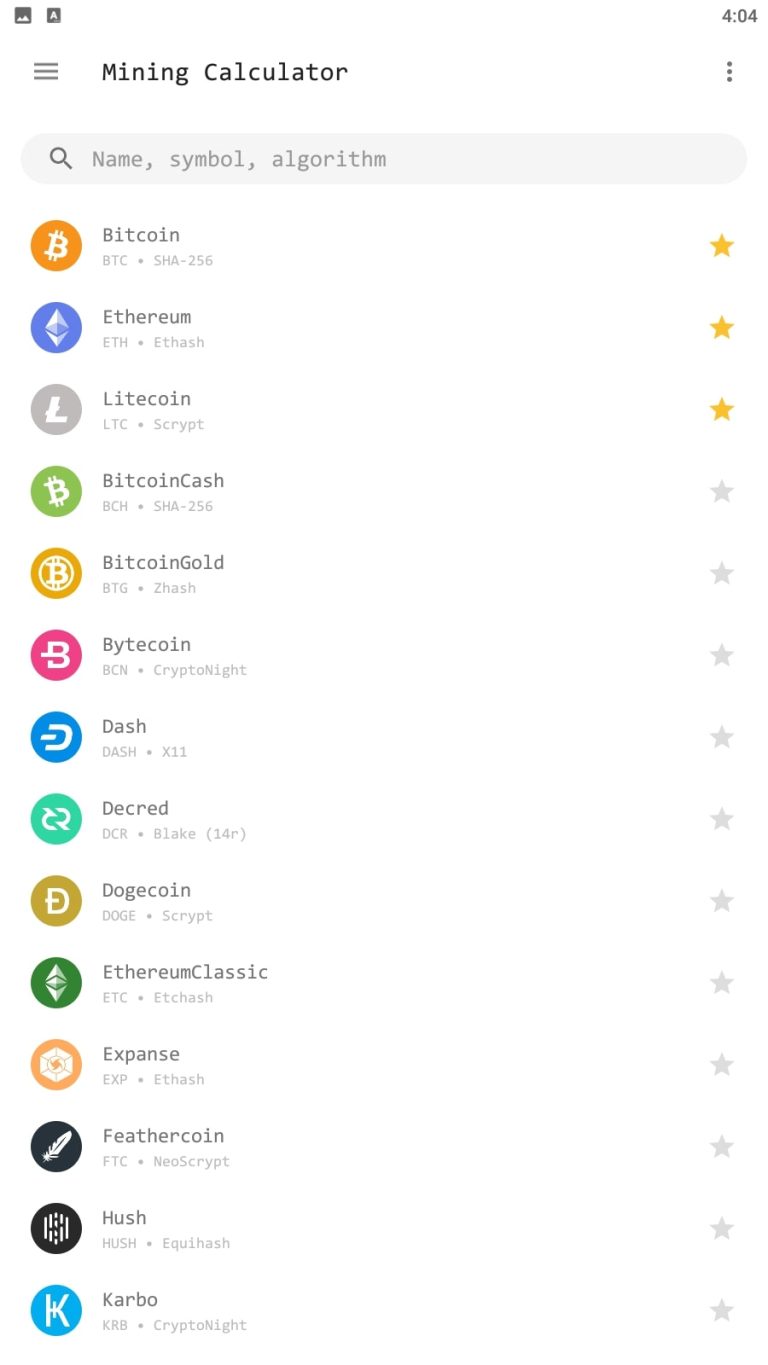A detailed, cleaned-up caption for the image could be:

---

This image appears to be a screenshot of a cryptocurrency website, displaying a list of various cryptocurrencies along with their symbols and algorithms. The screenshot is set against a black background with grey text, making the details stand out.

At the top-left corner of the image, there are two square icons, followed by the text "404" on the right, indicating an error or status code. Alongside this, on the right, there is a hamburger menu icon, and below it on the left, a "Mining Calculator" label is present with three buttons on its right side. A search bar is also visible, containing the placeholder text "Name Symbol Algorithm."

Below the search bar, a list of cryptocurrencies is displayed, each with its corresponding symbol and algorithm. The cryptocurrencies featured include:

1. **Bitcoin (BTC)**: An orange Bitcoin symbol with SHA256 algorithm, denoted by a highlighted yellow star.
2. **Ethereum (ETH)**: A blue Ethereum icon with ETHASH algorithm, also marked by a yellow star.
3. **Litecoin (LTC)**: A grey Litecoin symbol with SCRYPT algorithm, paired with a yellow star.
4. **Bitcoin Cash (BCH)**: A green icon alongside SHA256 algorithm, with a grey star.
5. **Bitcoin Gold (BTG)**: A yellow icon with ZASH algorithm, accompanied by a grey star.
6. **ByteCoin (BCN)**: A deep pink icon with CRYPTOLITE algorithm, grey star next to it.
7. **Dash (DASH)**: A blue circle icon with X11 algorithm, and a grey star.
8. **Decred (DCR)**: Green circle symbol featuring BLAKE 34C algorithm, with a grey star.
9. **Dogecoin (DOGE)**: A greenish-yellow circle with SCRYPT algorithm, paired with a grey star.
10. **Ethereum Classic (ETC)**: A green circle icon with ECHTASH algorithm, and a grey star.
11. **Expanse (EXP)**: An orange circle depicting ECHTASH algorithm, grey star.
12. **Feathercoin (FTC)**: A black circle with a feather symbol and NEOSCRYPT algorithm, shown with a grey star.
13. **HUSH (HUSH)**: A black circle with white lines and dots, running EQUAL HASH algorithm, with a grey star.
14. **Karbo (KRB)**: Blue circle marked with a "K" and CRYPTOLITE algorithm, sporting a grey star.

---

This caption provides a comprehensive description of the visual and textual elements present in the screenshot, ensuring that even those unfamiliar with cryptocurrency can understand the context and details.